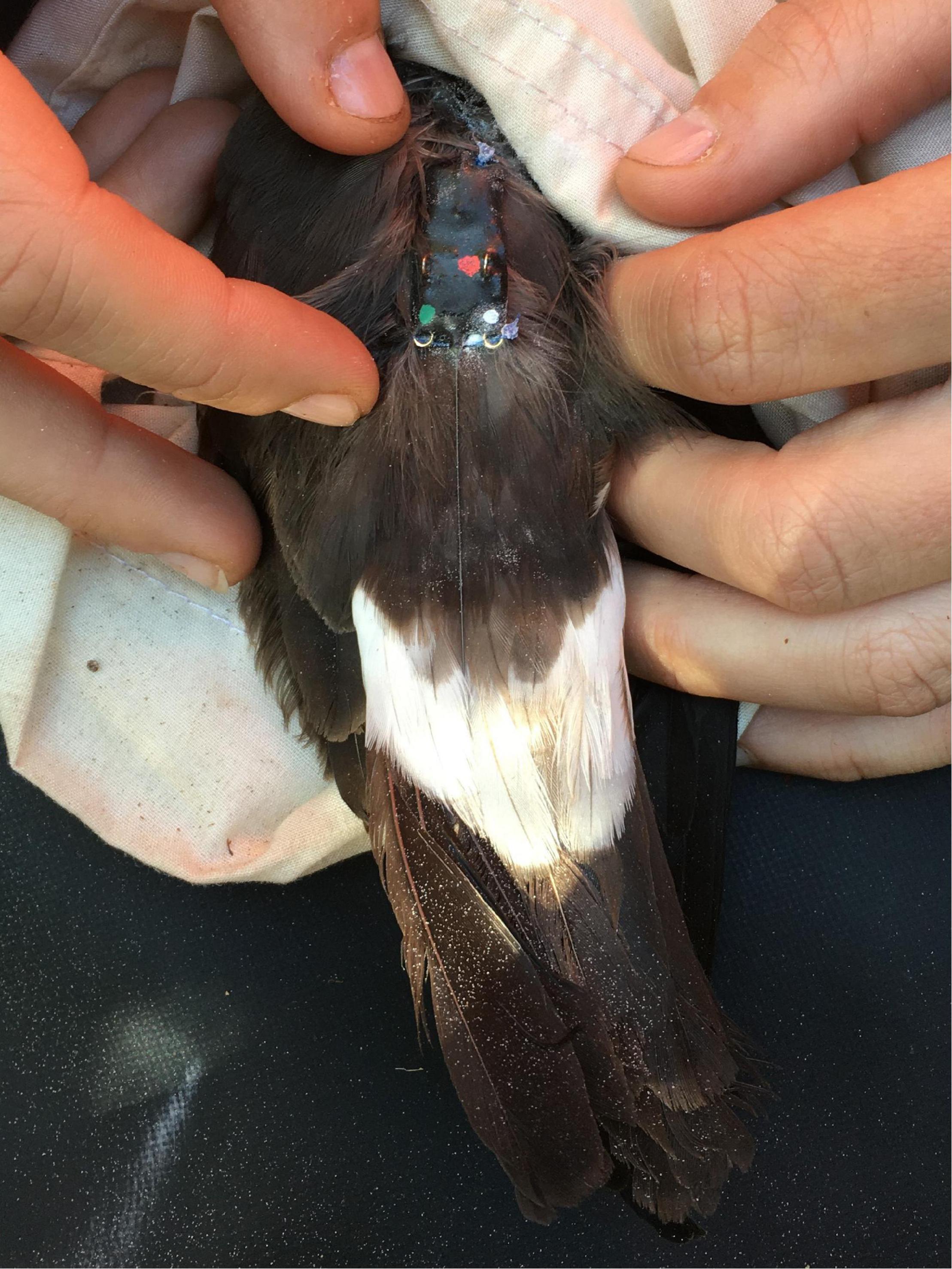This detailed photograph captures a close-up view of a pair of Caucasian hands carefully holding and spreading the feathers of a bird. The bird, whose head is burrowed into a white, burlap-like cloth, exhibits a composition of brown plumage with a distinct layer of white feathers adorning its center. Its tail, predominantly black with small white spots, extends toward the bottom of the image. Upon spreading the bird's feathers, a section of leathery black skin becomes visible, adorned with multicolored dots in red, green, and white, as well as silver or brass rings, though it remains uncertain whether these are natural markings or part of an applied device. The bird rests on a black surface, dotted with tiny white spots, adding contrast to the scene. The hands, shown only by their fingers, appear to be gently revealing the bird's intricate and colorful skin beneath the feathers and the enveloping white cloth.